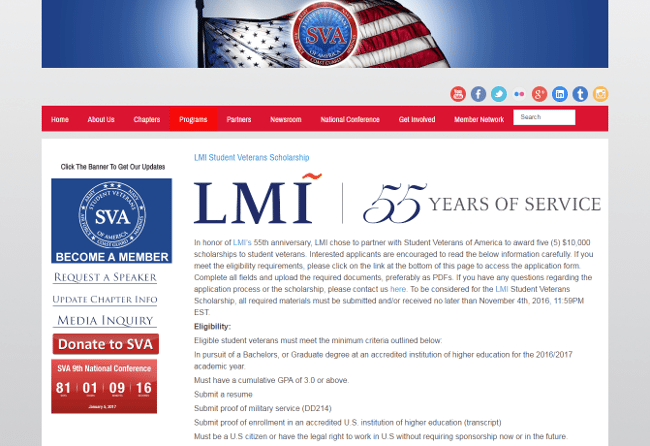This screenshot, taken from a notably patriotic website, features a dark blue bezel on both the left and right sides, each adorned with an American flag. The flag itself displays a blue canton on the left and alternating red and white stripes on the right, all attached to a dark black pole. Central to this flag is an animated circle with three sections: an outer white ring, a middle red ring, and an innermost blue circle, accompanied by the red text "SVA" at the top.

Below the flag, there is a section with a gray background displaying icons for various social media platforms, including YouTube, Facebook, Twitter, Instagram, Google Hangouts, and LinkedIn. Further down, a dark red bezel contains navigation options such as "Home," "About Us," "Chapters," and "Program"—the latter of which is highlighted in a blood-red color, indicating selection. Additional menu items listed are "Parameters," "News," "Newsroom," "National Conference," "Get Involved," and "Member Network."

Prominent on the page are the bold, dark blue letters "LMI," adjacent to which the number "55" is displayed in blue with the accompanying phrase "Years of Service" in gray.